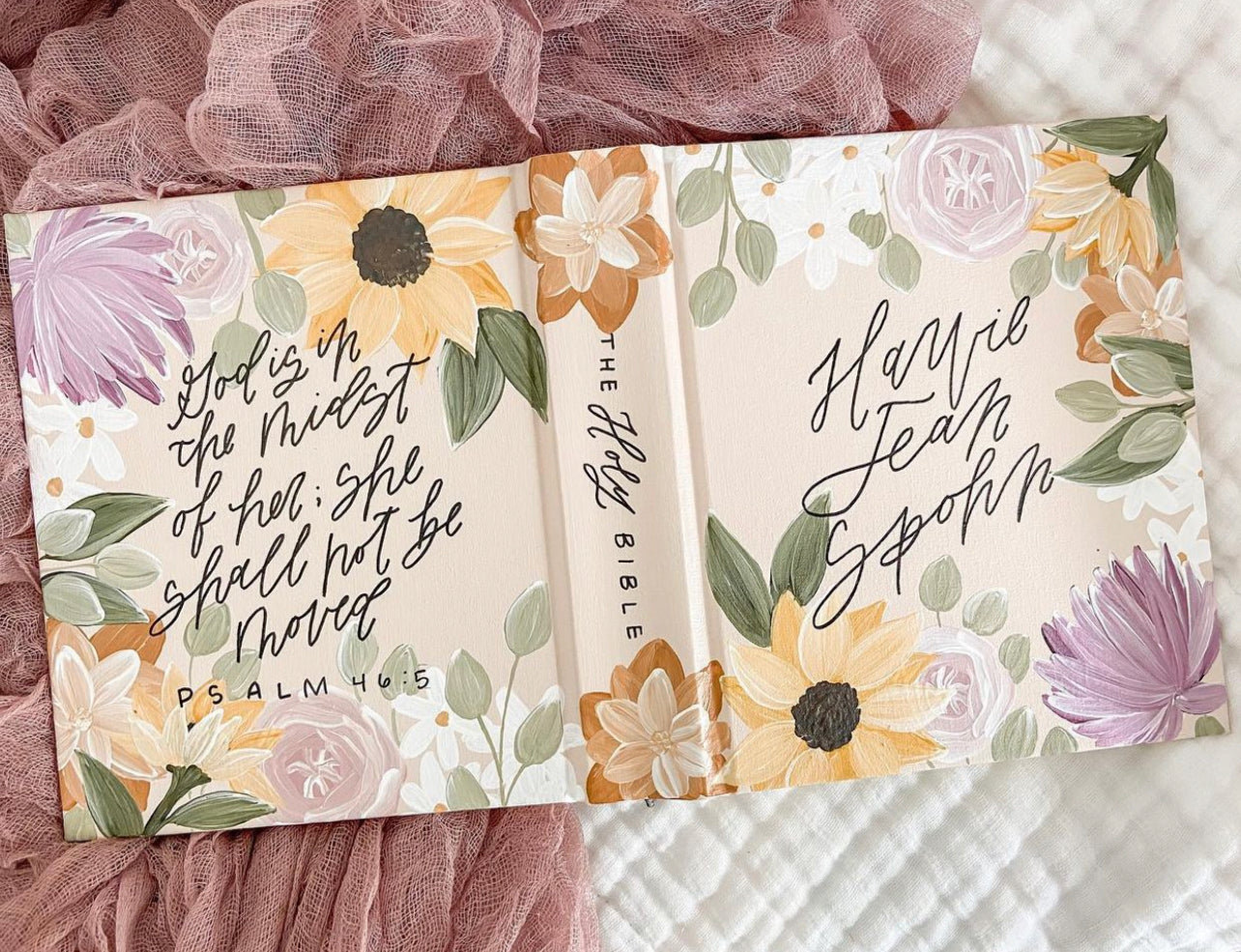The image is a detailed photograph of an open Bible resting on a surface adorned with pink gauzy material on the left and a white, fluffy coverlet on the right. The spine of the Bible clearly reads "The Holy Bible." The book's cover is predominantly white, decorated with illustrations of purple and yellow flowers accompanied by green leaves. Notably, the interior on the left page features a prominently displayed quote in cursive text: "God is in the midst of her. She shall not be moved. Psalm 46:5." The overall scene presents a serene and delicate composition, with the combination of soft textiles and floral motifs enhancing the spiritual and peaceful ambiance of the image.